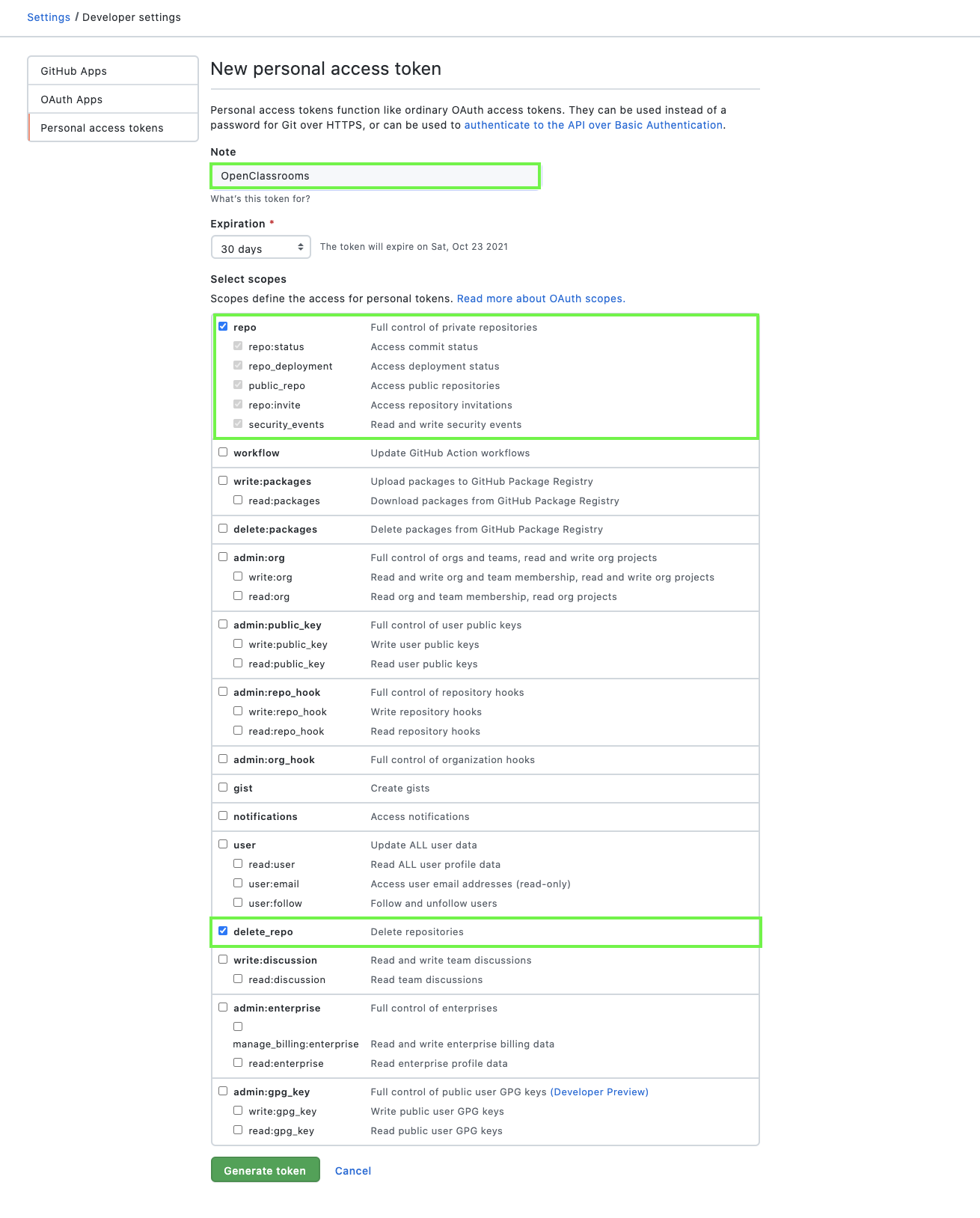**Descriptive Caption:**

The image depicts a setting screen for developer settings within a platform, likely GitHub. At the top left, the word "Settings" is displayed in blue, followed by "Developer settings" in black text, separated by a gray line. Below this, a small menu lists various options including "GitHub Apps," "OAuth Apps," and "Personal access tokens," with an orange highlight on the left.

The main column presents the title "New personal access token." Below this, a description explains that personal access tokens function like ordinary OAuth access tokens, serving as an alternative to a password for Git over HTTPS or for authenticating to the API over basic authentication.

Further down, a green box notes "Open classrooms." Next is a section titled "What's this token for?" followed by an "Expiration" section marked with a red asterisk, and a textbox indicating "30 days." It notes that the token will expire on Saturday, October 23rd, 2021.

The section "Select scopes" invites users to define the access for personal tokens, with a link in blue text to read more about OAuth scopes. A series of checkboxes with descriptive labels follows:
- "repo" with a blue checkmark, allowing full control of private repositories.
- Several unchecked boxes for "repo:status" (Access commit status), "repo_deployment" (Access deployment status), "public_repo" (Access public repositories), "repo:invite" (Access repository invitations), and "security_events" (Read and write security events).
- Other scopes listed include "workflow", "write:packages", "delete:packages", "admin:packages", "admin:public_key", "admin:repo_hook", "admin:org_hook", "notifications", "user", "delete_repo" (checked), "write:discussion", "admin:enterprise", and "admin:gpg_key."

At the bottom left of the screen is a green button labeled "Generate token," and beneath it, the text "Cancel" in blue.